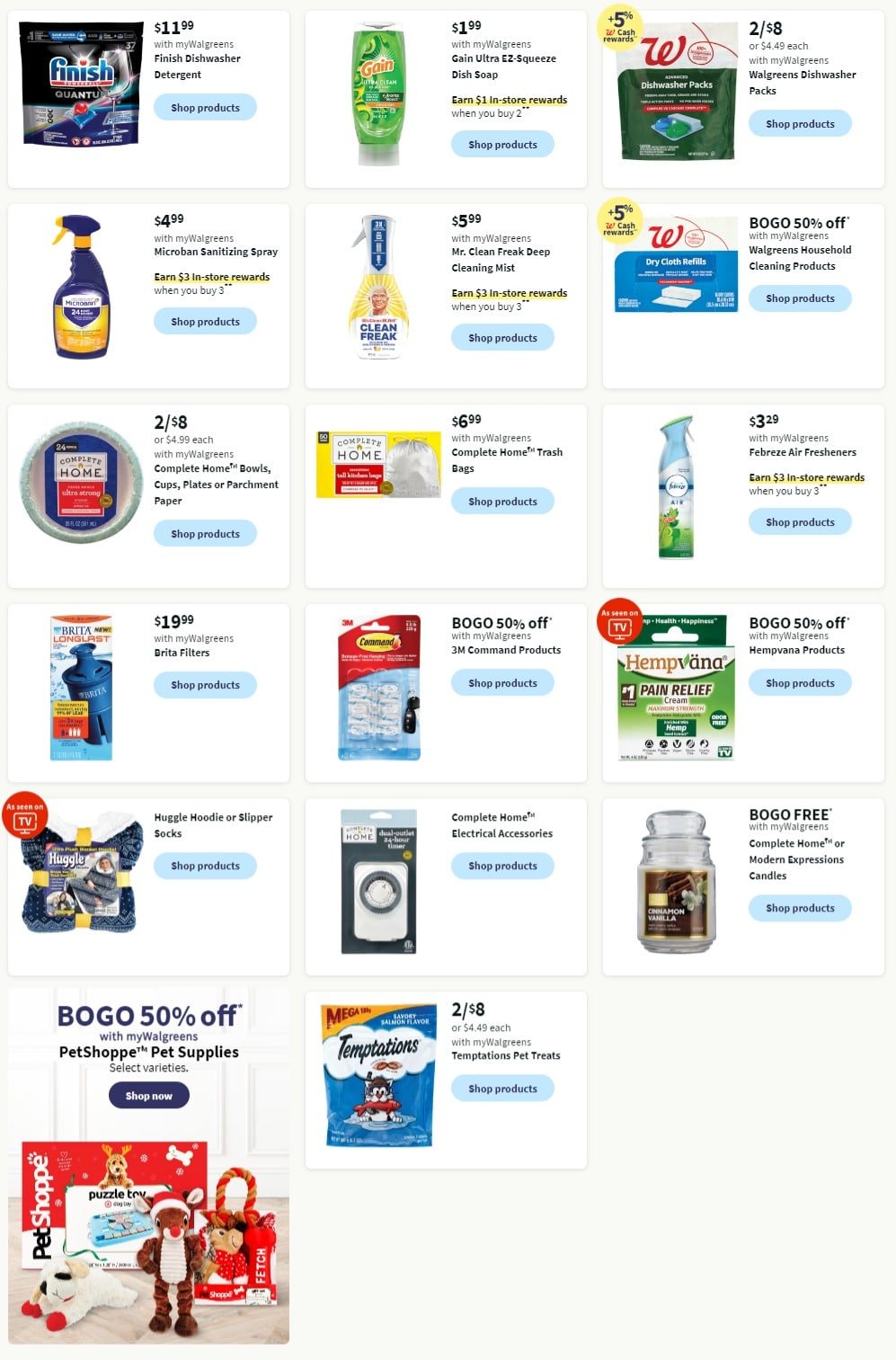This image showcases a digital weekly ad page from Walgreens, featuring various housewares and cleaning products. The backdrop is a light gray, adorned with numerous white boxes, each containing different product listings. Products like Finish dishwasher detergent, Gain Ultra Easy Squeeze dish soap, and Walgreens dishwasher packs are prominently displayed. A variety of sprays, paper plates, trash bags, and Febreze are also included. Noteworthy promotions such as "BOGO 50% off" on Command strips and "BOGO free" on Complete Home or Modern Expression candles stand out.

Each product listing includes different pricing structures, ranging from regular prices to special sales and BOGO deals. In the bottom left corner, a small ad highlights a "BOGO 50% off" offer on select pet supplies with a link to shop now, branded with "MyWalgreens Pet Shop."

The entire page has a Christmas theme, suggesting it was published during the holiday season. Its design is simple yet effective, featuring black text, subtle gray drop shadows, and straightforward product images.